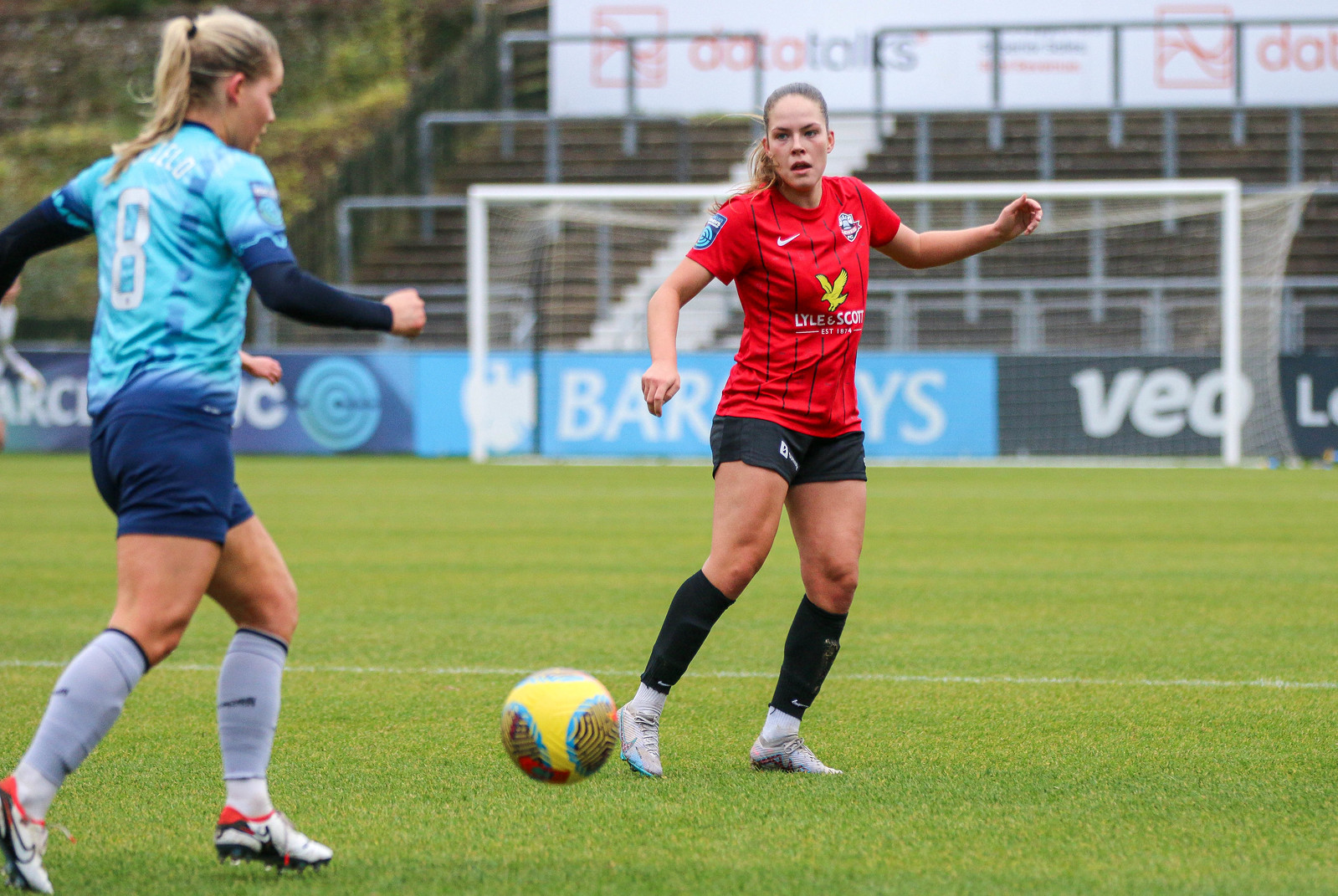In this image, two female soccer players from opposing teams are captured in mid-action on a green grass soccer field marked with multiple white lines. The player in the foreground, dressed in a light bluish-green jersey with navy shorts, appears poised to kick the ball, adorned with a colorful design featuring orange, yellow, blue, red, and zebra stripes. Her opponent, wearing a red jersey with black shorts, is either preparing to defend or intercept the ball, which is slightly airborne. In the background, the white goal with its matching net stands empty, suggesting a practice session, while empty bleachers rise behind it, separated from the field by a railing draped with blue and black banners. The banners and distant white billboard, marked with out-of-focus orange and blue logos reading "Data Talks," contribute additional depth to the scene. Additionally, the railing on the far right side bears the letters "VEO" in white, further adding to the detailed setting of this dynamic athletic moment.